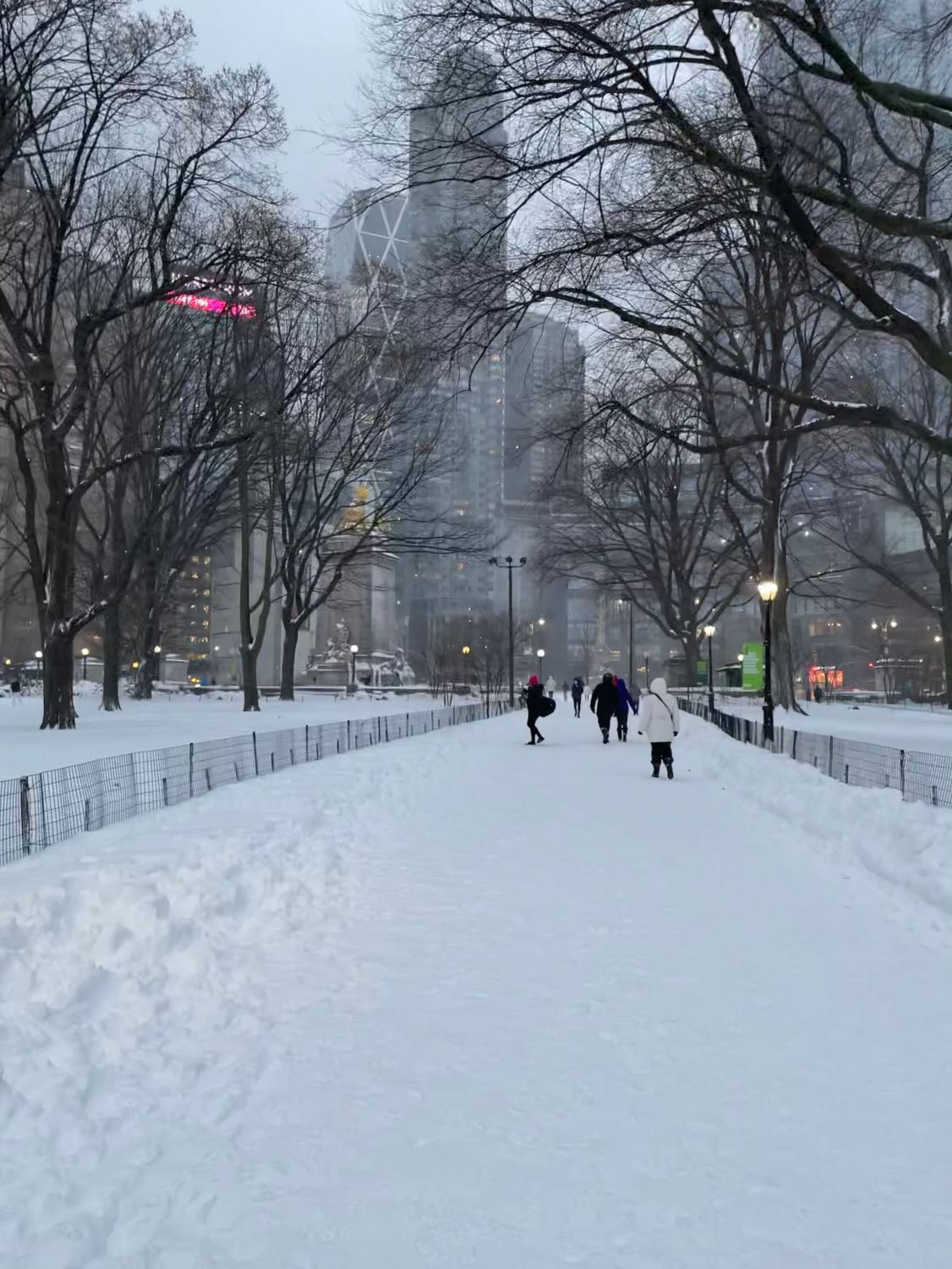This image captures a snowy park pathway in the midst of an urban environment, likely in a major city such as New York or Hong Kong. The snow-covered path, estimated to be around two to four inches deep, winds through the park, flanked by trees barren of leaves due to the winter season. A small metal mesh fence runs along the edges of the path, separating the walkway from the tree-lined areas. 

In the center of the image, several people are strolling along the snow-laden path, bundled up in winter attire including heavy coats, boots, gloves, and hats. Notably, one individual is dressed in a white parka with the hood pulled up, while others wear wool caps and different colored outfits, including a noticeable black outfit paired with a red hat.

Surrounding the park, towering, modern skyscrapers dominate the backdrop, their windows illuminated against the hazy, gray afternoon sky, suggesting a recent snowfall. To the left of the image, a large statue is visible in the distance, adding to the sense of a central city park. Street lamps are positioned along the right side of the photo, casting light over the snow and highlighting the path that tapers off into the urban cityscape. Signs and additional distant figures populate the background, reinforcing the scene’s urban nature.